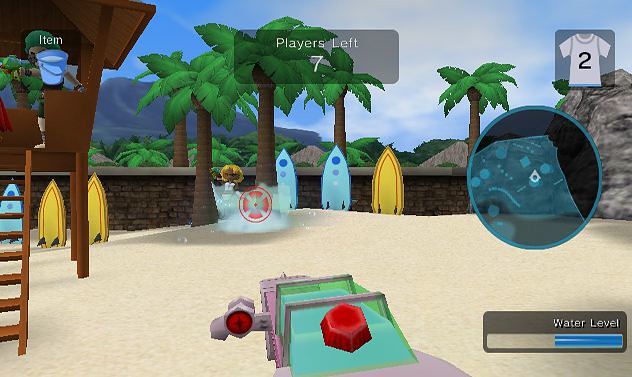The image appears to be a still shot from a video game set in a warm, coastal environment. The focal point of the scene is a beach where five surfboards are standing upright in the sand: two are blue and three are yellow. Pine trees in the background suggest a warm climate. At the top center of the image, there is an indicator reading "Players Left: 7." To the top right, a white t-shirt icon with the number "2" is displayed. On the top left, an icon of a bucket labeled "Item" is visible. In the foreground, facing towards the surfboards, is an unidentified vehicle. The lower right portion of the screen features a "Water Level" gauge, which is approximately half full with a blue color. On the left side of the image, there is a raised platform accessible by a ladder.